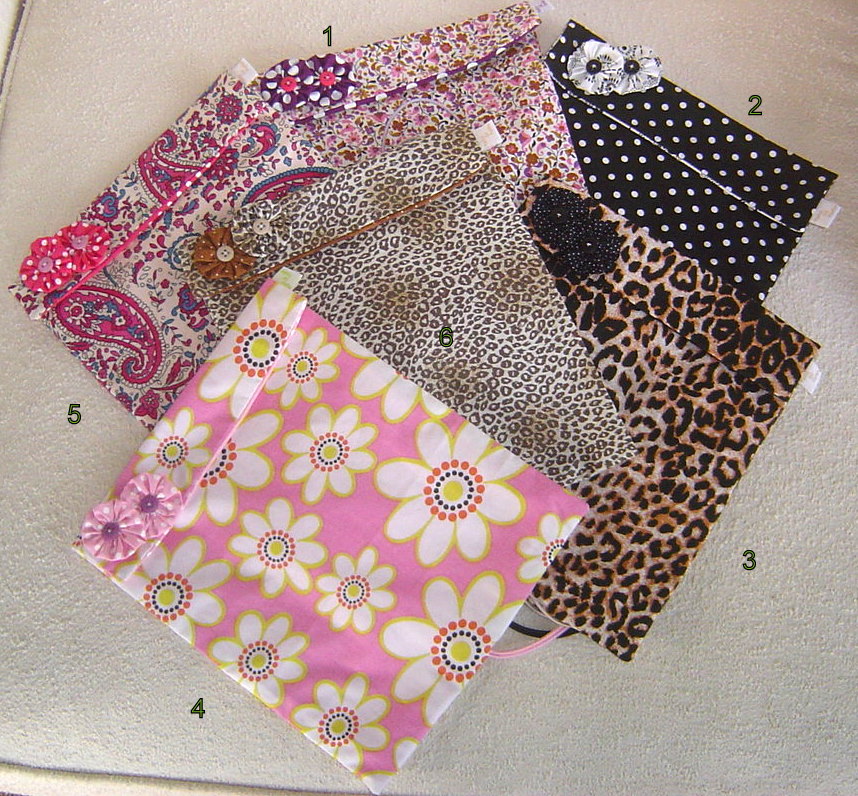The image depicts six small fabric pouches laid out on a beige couch cushion, showcasing a neat arrangement slightly overlapping one another. They are all numbered from one to six in black numerals. Each pouch has a distinctive design and two appliqué fabric flowers with coordinating buttons on the top flap as a decorative closure.

Starting from the left:
1. A blue, white, and pink paisley pouch with fabric flowers that have pink polka dots and lighter pink buttons.
2. A brown, pink, and white floral design pouch adorned with purple polka dotted flowers and pink buttons.
3. A black pouch with white polka dots, featuring white flowers inscribed with black text and black buttons.
4. A leopard print pouch with black polka dotted flowers and black buttons.
5. An animal print pouch with one matching fabric flower and another brown with white polka dots and white buttons.
6. A pink pouch decorated with yellow, white, orange, and blue flowers, highlighted with pink flowers adorned with white polka dots and purple buttons.

Each pouch also contains a small square tag sewn into its side. The fabric flowers appear slightly varied in color and pattern, adding a cohesive yet distinct visual appeal to each piece. The tactile quality of the handcrafted pouches suggests they are ideal for holding small trinkets or personal items, akin to a slim, soft, square-shaped purse. The beige couch cushion's corded border is visible at the bottom left of the image, emphasizing the casual, cozy setup of this homemade display.